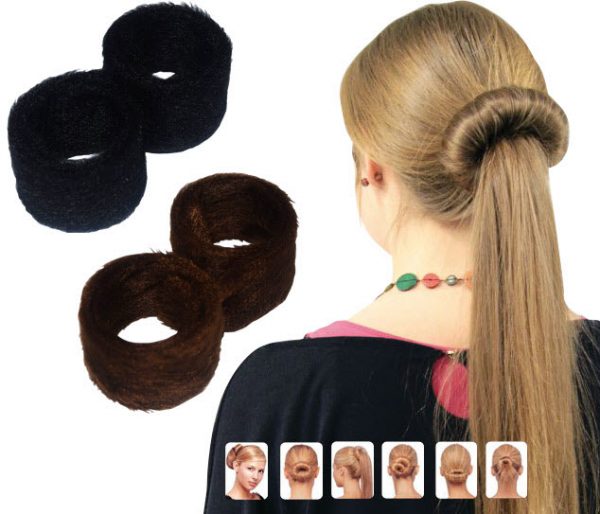This image, likely from a website advertising a hair styling product, features a versatile hair accessory that facilitates creating buns and ponytails. Set against a plain white background, the top left corner displays two black cuff-like objects, each about two inches tall, and two dark brown ones below them. To the right, the back of a young woman’s head showcases her long, thin blonde hair styled into a partial bun using one of these accessories. She wears a dark pink shirt layered with a black jacket and a multicolored necklace, with a notable earring visible. Beneath her, six images demonstrate various hairstyles achievable with the product, including a complete bun, a high ponytail, and different bun designs viewed from multiple angles. This detailed presentation highlights the product's versatility and practical application in everyday hair styling.